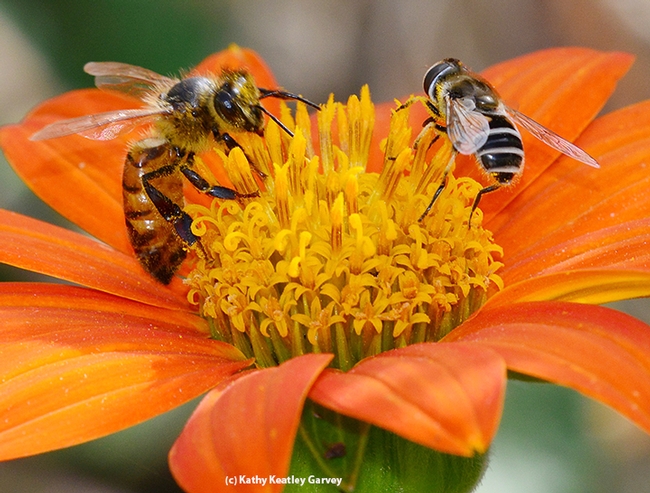This detailed close-up image features two bees extracting nectar from an orange-petaled flower. The flower's prominent central pistil, adorned with numerous yellow, straw-like structures, serves as a focal point for the bees' activity. Positioned on the left side, a larger bee with a distinguishable almost wasp-like appearance showcases a golden-yellow abdomen with black stripes, longer black legs, and clear wings. On the right side, a smaller bee displays a black abdomen with white stripes and transparent wings. Both bees are engrossed in collecting pollen. The background of the image is artistically blurred, accentuating the vivid details of the flower and bees. At the bottom center of the image, the stem of the flower can be spotted peeking beneath the vibrant petals. The photo is credited to Kathy Keatley Garvey.